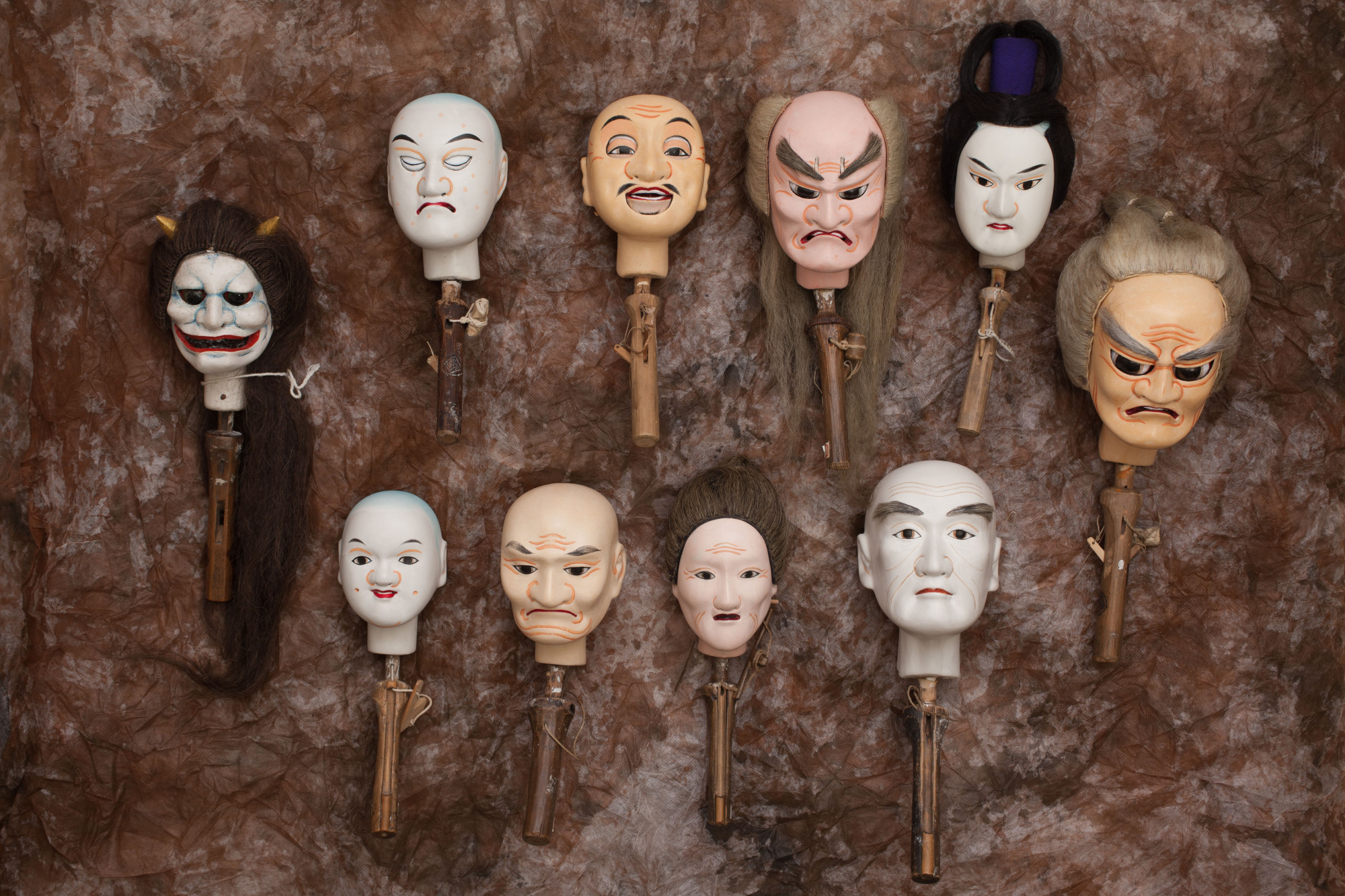The image depicts a collection of 11 intricately crafted puppet heads, each representing different ages and genders, with a distinctly Asian aesthetic. Arranged neatly on a red and white table, except for the heads on the far left and far right, these puppets include male, female, and child figures, as well as representations of older individuals. The heads vary in their hair styles—some are bald, while others have varying shades of hair. Notably, the puppet head on the far right has gray hair and large eyebrows, and the one on the far left features brown hair and a notably white face.

The puppet heads are mounted on sticks that likely serve a functional purpose, possibly to operate the puppets or to attach them to larger bodies. The photograph captures these heads from a top-down perspective, emphasizing the detailed craftsmanship and the eerie, expressive faces of the puppets. The background is a brown and gray wall, which adds a somber tone to the image. Some of the faces are scary and evoke strong emotions, with details like a witch-like face with horns and a mean-looking male with a tuft of hair and frowning eyebrows. The puppet heads form an oval shape, creating a visually striking arrangement that draws attention to the diverse expressions and intricate details of each head.